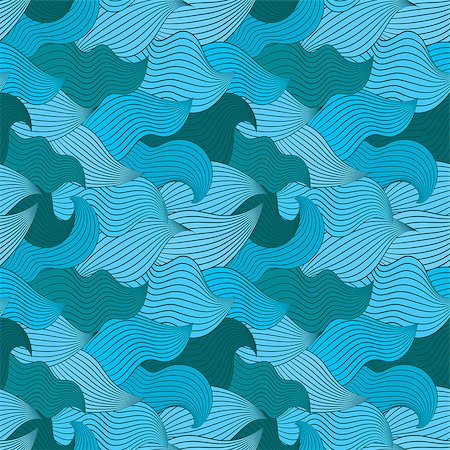The image features an abstract depiction of blue and green wavy swirls, resembling the pointed hair on a troll. These swirls are represented in various shades, ranging from baby blue and Carolina blue to darker hues such as navy and turquoise. Interspersed among these are green swirls in hues from a light powder green to a deep forest green, though the blue swirls are more prominent. The swirls are densely packed with lines, potentially in navy blue or black, that trace the curves and enhance the wavy texture. The swirls point in multiple directions, predominantly towards the right, creating a sense of turbulent motion. With its complex, freeform arrangement, the image gives an impression of dynamic movement and could serve as a striking visual pattern, possibly for wallpaper or another decorative surface. The lack of text and the vibrant interplay of colors contribute to its abstract, painterly quality.